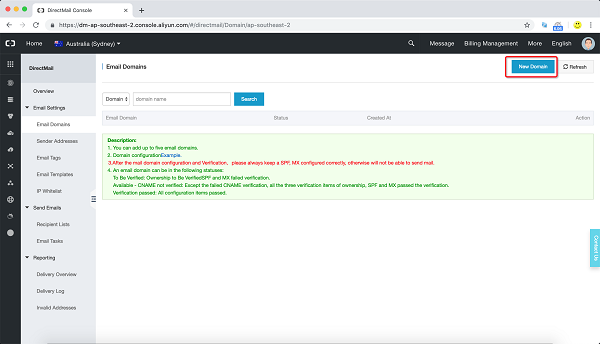A screenshot of a web console interface tailored for managing email domains. The top section labels the console as "Decimal Console" and features navigational links for Home, Messages, Billing Management, Help, and a Language Selector set to English. On the top right side, a search bar and a prominent "New Domain" button, highlighted in blue, stand out. A left sidebar provides detailed navigation options including Overview, Email Briefings, Email Addresses, Email Reports, Senders, Email Tasks, Delivery Reports, Inbound Domains, and Settings.

The main content area is dedicated to Email Domains, featuring another search bar specifically for domain names and a green box containing essential instructions and descriptions regarding email domain setup. Users can add up to five email domains, configure these domains as senders, and need to ensure proper configuration of SPF and MX records after domain addition and verification. If verification fails, users are instructed to check ownership, SPF, and MX records.

The primary table in the main content area has columns for Email Domain, Status, Created At, and Action, though it currently lists no domains. A refresh button is conveniently located next to the "New Domain" button, allowing users to update the view easily. The interface is designed with a clean, structured layout that emphasizes functional navigation and efficient management of email settings.